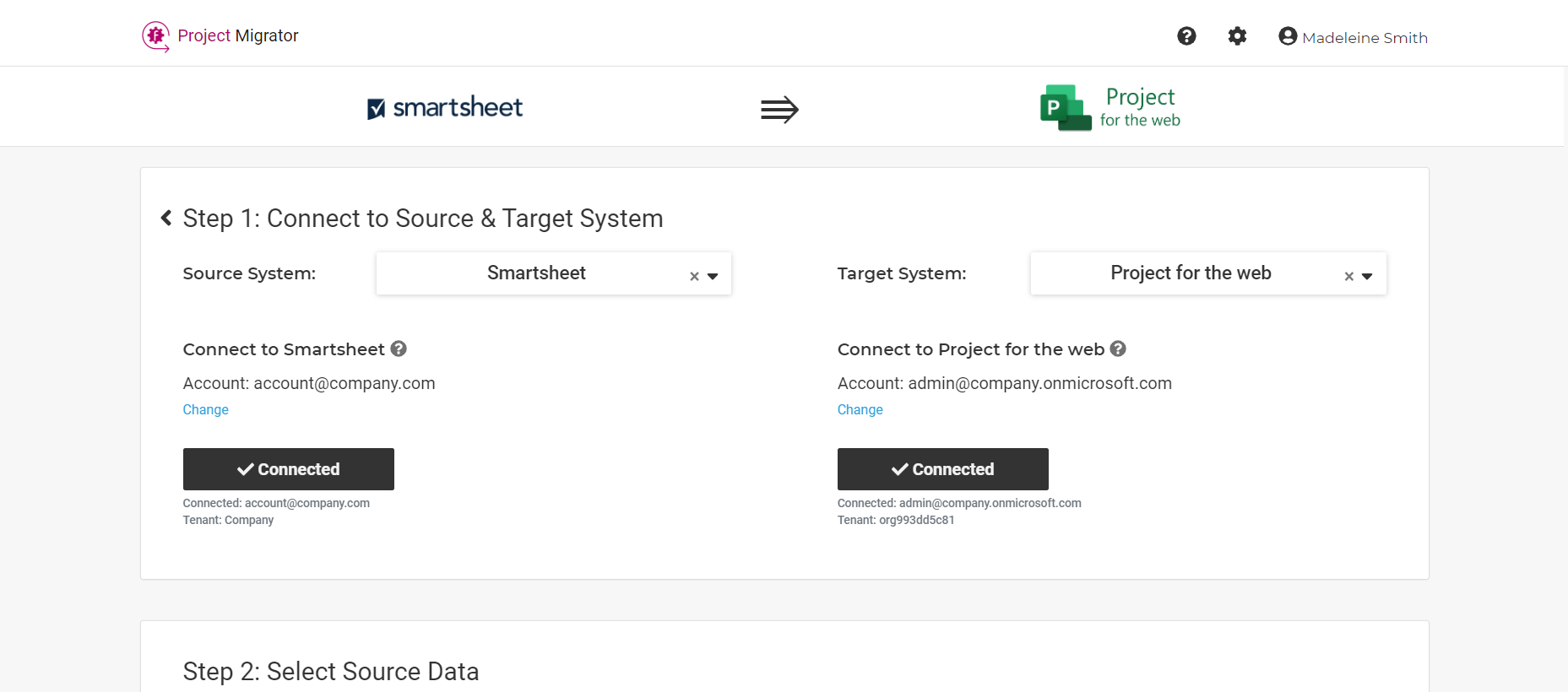The image depicts a computer screen displaying a user interface for a software application called "Project Migrator." In the upper right-hand corner, there is a profile picture of a user named Madeline Smith. On the left side of the screen, the application name "Project Migrator" is prominently displayed. The main focus of the screen is on two sections indicating the progress of a migration process. 

At the center of the interface, an arrow points from the Smartsheet logo on the left to the Microsoft Project icon on the right, symbolizing the migration from Smartsheet (the source system) to Project for the Web (the target system). Below this, there are two boxes, each labeled "Connected" with a check mark, indicating a successful connection to both the source and target systems.

The instructions for the migration process are clearly divided into steps. The visible steps are:
1. "Connect to source and target system," with the source being Smartsheet and the target being Project for the Web.
2. "Select source data," which is the subsequent step in the migration process.

The user interface is predominantly white, with minimal use of color to highlight specific icons and elements, creating a clean and functional layout.